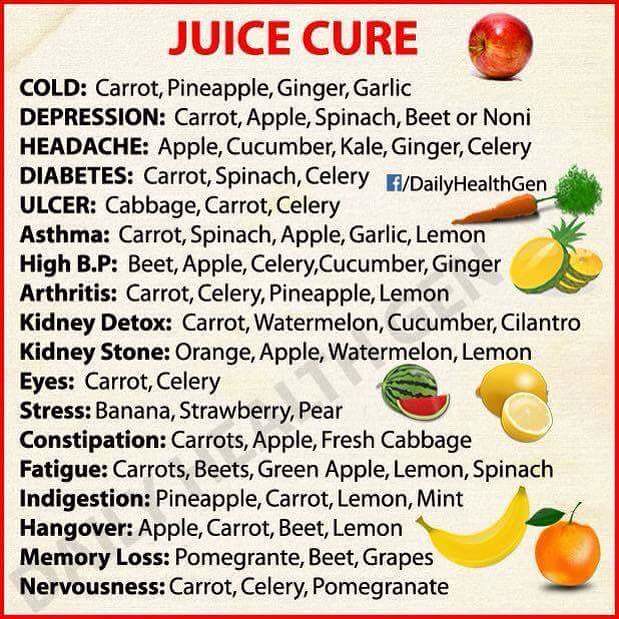The image has a tan, beige-pink background framed with a vivid red border, and is titled "Juice Cure" in prominent red text at the center top. Adjacent to the title is an image of an apple. The core content of the image includes multiple lines of black text listing various health conditions alongside recommended fruit and vegetable juice combinations to alleviate those conditions. Starting from the left, the conditions listed in bold black text are: cold, depression, headache, diabetes, ulcer, asthma, high blood pressure, arthritis, kidney detox, kidney stone, eyes, stress, constipation, fatigue, indigestion, hangover, memory loss, and nervousness. Each condition is paired with a blend of fruits and vegetables suggested to cure it; for example, 'cold' features carrot, pineapple, ginger, and garlic, while 'depression' recommends carrot, apple, spinach, beet, or noni. Along the right side of the image are pictures of various fruits, complementing the textual content and providing a visually appealing contrast.